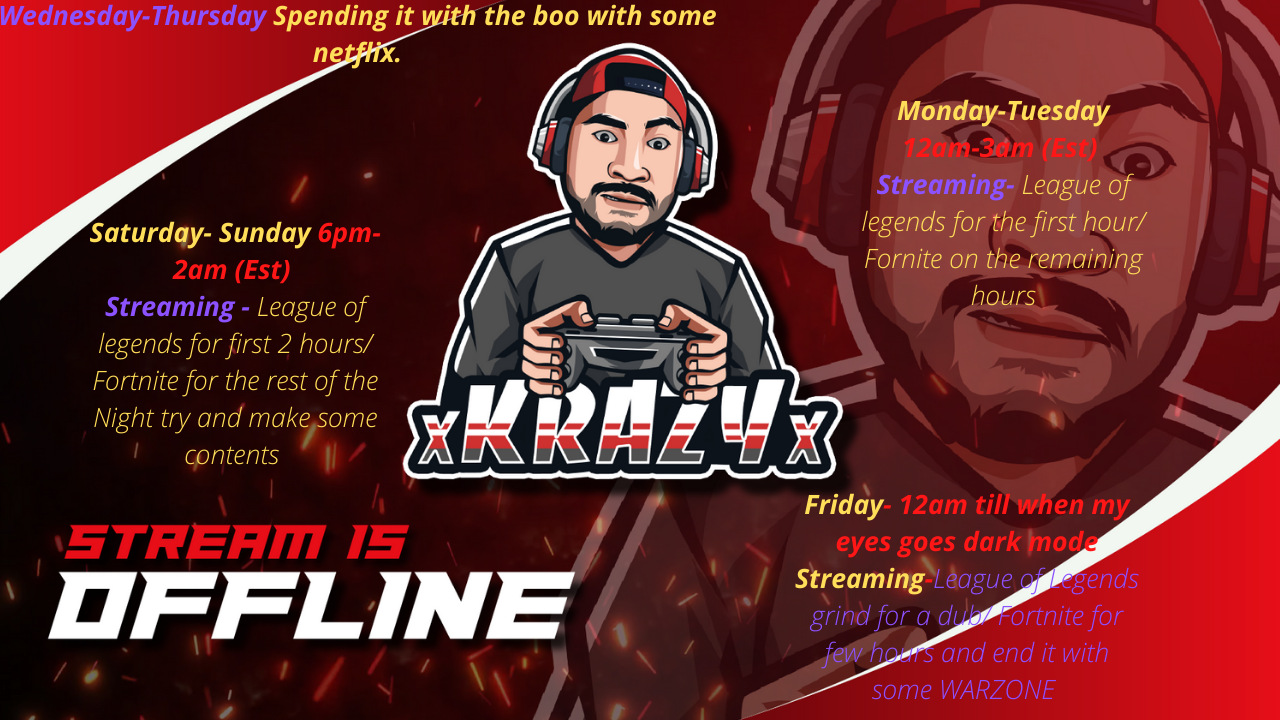This advertisement banner for the streaming schedule of the individual known as XKRAZYX features a detailed colored pencil graphic of an Asian man, who is depicted wearing a gray long-sleeved shirt with white stripes, headphones, and holding a gaming controller. He has a mustache and beard. His name, XKRAZYX, is prominently displayed below his image, and the graphic is outlined in white. The image is framed with red diagonal corners, accented with white inward stripes. The banner is packed with various texts detailing the streaming schedule, but its busy layout makes it challenging to read and engage with effectively.

The schedule details are as follows:

- **Monday through Tuesday (12 a.m. to 3 a.m. EST)**: Streaming starts with *League of Legends* for the first hour, followed by *Fortnite* for the remaining hours.
  
- **Wednesday through Thursday**: Engaging in Netflix sessions with their significant other ("boo").
  
- **Friday (12 a.m. until eyes go into dark mode)**: Streaming *League of Legends* for an unspecified duration, then *Fortnite* for a few hours, and ending the session with *Warzone*.

- **Saturday through Sunday (6 p.m. to 2 a.m. EST)**: Streaming *League of Legends* for the initial two hours, followed by *Fortnite* to create content for the rest of the night.

In the lower left-hand corner, there's a notification indicating the stream is currently offline, as denoted by the bold italic text "offline" in white. Despite the high-quality image and the wealth of information, the organization of text could use significant improvement for better legibility and user engagement.